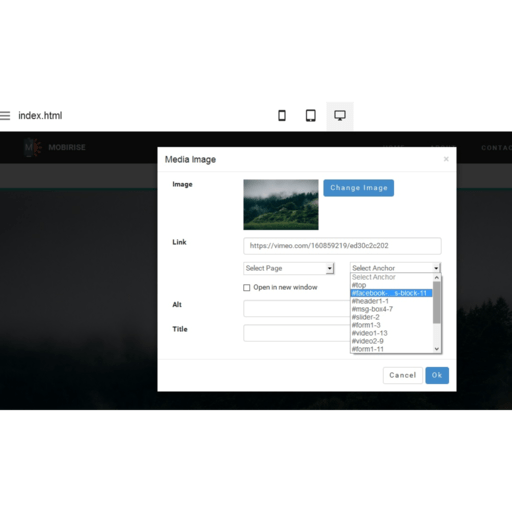The image showcases a user interface on a black background. At the top, "index.html" is prominently displayed alongside a hamburger icon. The interface includes icons representing a phone, tablet, and computer, with the computer icon highlighted in gray. Below, there's a media section that features an image of grass. Next to it, a blue rectangle button with white text reads "Change Image." 

The interface also includes options for links, with notable elements such as a "Select Page" dropdown and a checkbox for "Open in a New Window." Additionally, there are multiple "Select Anchor" options and a list of items, one of which is highlighted in blue. A scroll bar is present, indicating more items in the list. 

Towards the bottom, a white rectangle contains a "Cancel" button in black, as well as a blue rectangle with the word "Okay" in white. There are fields labeled "ALT" and "Title," each with corresponding input boxes.